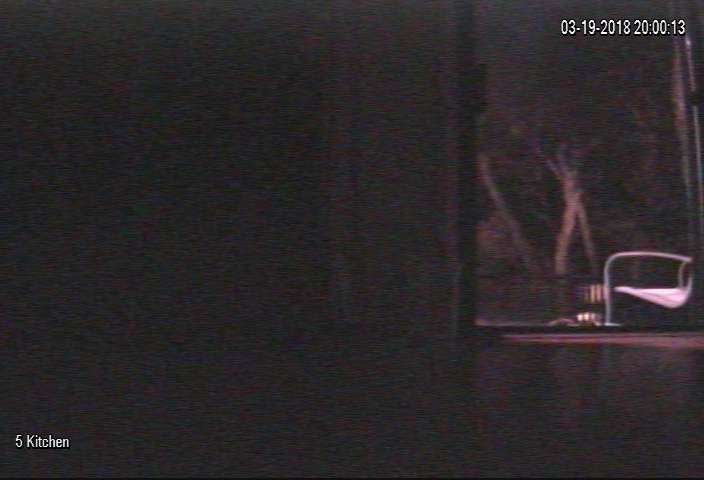This photograph, captured by a security camera, is a very dark and grainy image with a slight pink hue, making details hard to discern. In the top right corner, a timestamp in white font reads "03-19-2018 20:00:13." The bottom left-hand corner also in white font, states "5 kitchen." The majority of the image, particularly from the middle to the left side, is completely black and dark brown. On the right side, through an open door, an exterior view reveals what appears to be trees, possibly forming a forest scene. Some viewers suggest they see a hammock or a metal stand with something white hanging from it, while others mention the possibility of an alien-like creature among the trees. Inside the room, it is nearly pitch black, though there is a faint, bright object on the right side, which might be part of a chair. Overall, the image is too dark and blurred to identify any elements with certainty.